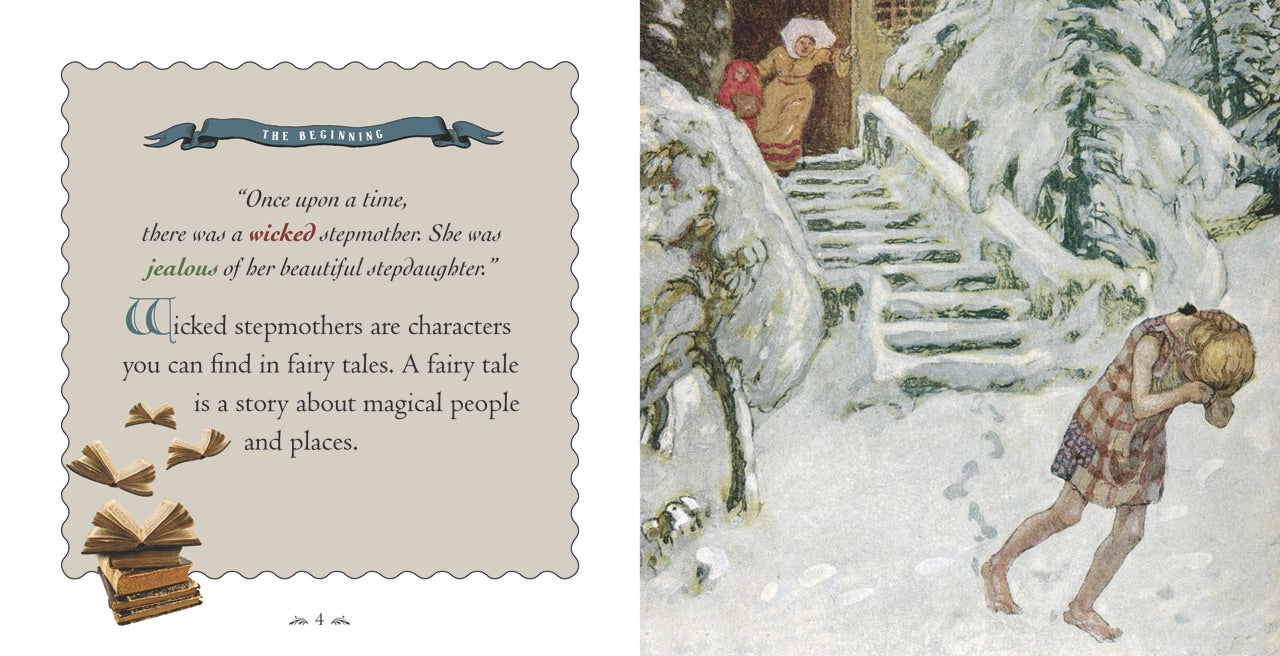The composite image is divided into two sections. The left section, set against a gray background with rigid, stamp-like edges, features a blue banner at the top that reads "The Beginning." Below the banner, three lines of black writing state: "Once upon a time, there was a wicked stepmother. She was jealous of her beautiful stepdaughter." Following this, four more lines of black writing explain: "Wicked stepmothers are characters you can find in fairy tales. A fairy tale is a story about magical people and places." In the bottom left corner of this section, there's an illustration of a stack of books.

The right section of the image depicts a colorful drawing set in a snowy landscape. Central to this scene is a staircase that ascends and slightly curves to the left, leading to a house. In the doorway stands a woman clad in a brown coat with a white, furry hood, accompanied by a small child to her left. At the foot of the stairs, footprints navigate the snow, leading to a young girl in the bottom right corner. This girl, wearing a checkered dress, has short blonde hair and appears distressed, with her head buried in her hands as she crouches in the snow.